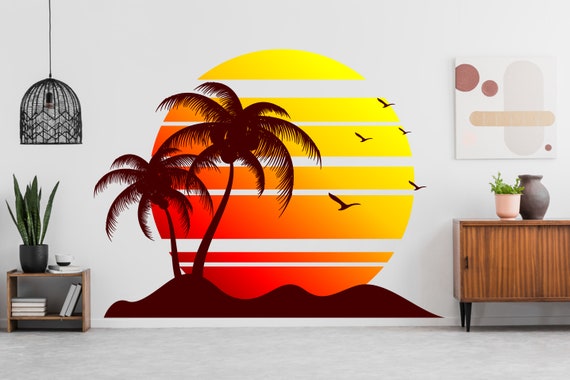This photograph captures the serene ambiance of an indoor living space. The focal point is a striking mural on a light grayish-white wall, featuring a large circular sun with a gradient from yellow to dark orange and horizontal lines with white spaces in between. The mural also includes two palm trees to the left, hills below them, and five seagulls flying in a V formation to the right. The floor is covered with light gray stone tiles, and there is white molding at the base of the wall. 

To the left of the mural, a black wicker hanging lamp descends from the ceiling above a small one-shelf wooden bookcase that houses an aloe plant in a black planter and a stack of books. To the right, there's a wooden side table with a cabinet beneath and two vases on top. Above this table, an abstract painting in beige and brown hues adorns the wall.

Overall, the room boasts a cohesive tropical theme, elegantly blending functional furniture with decorative elements to create a tranquil living area.